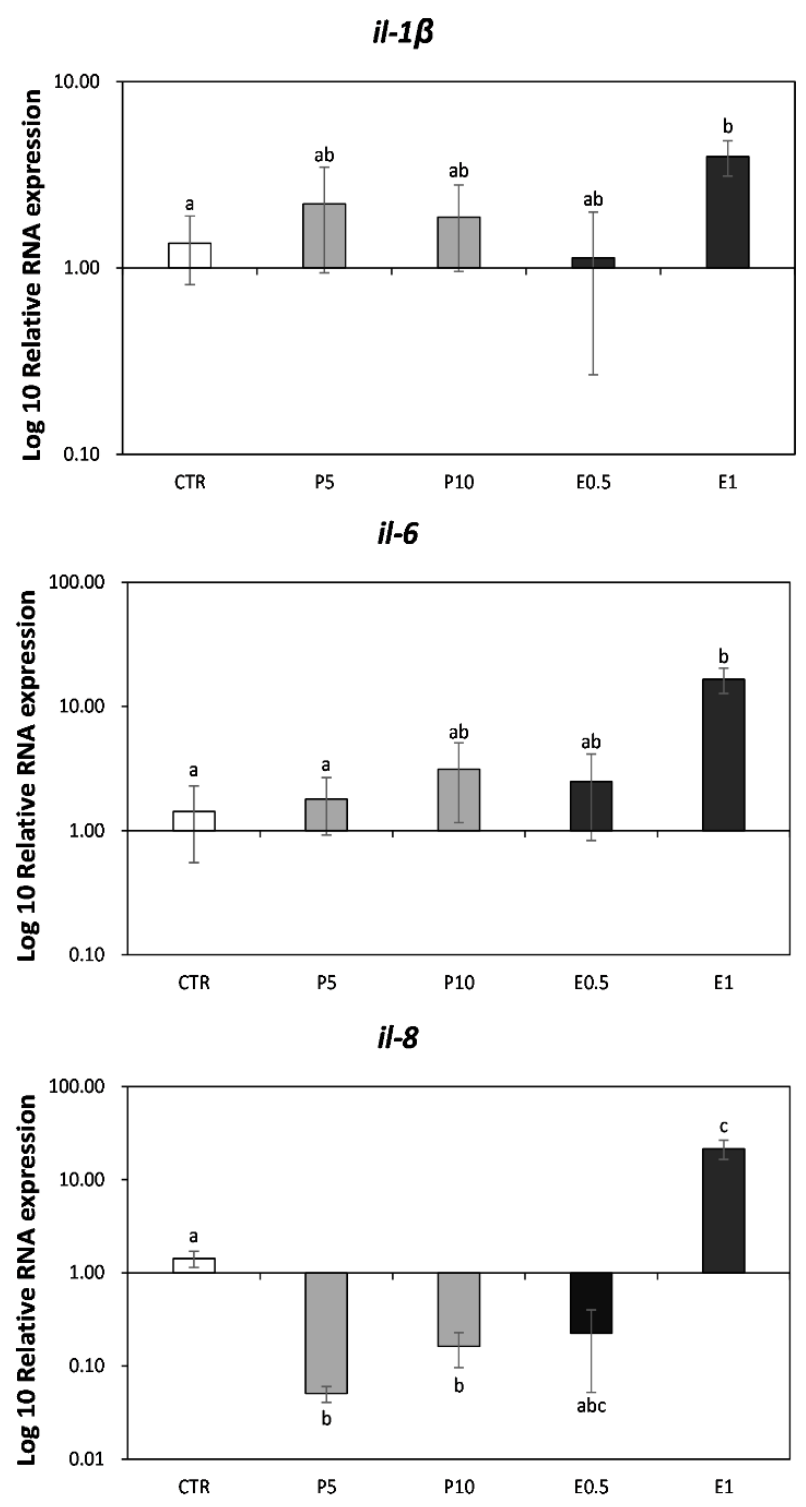This black and white image features three distinct bar graphs, each titled with log10 relative RNA expression on the y-axis and displaying data for different genes: IL-1B, IL-6, and IL-8. The x-axis for each graph is labeled with the categories CTR, P5, P10, E0.5, and E1, representing various experimental conditions or time points. The data points in the graphs are neatly organized, providing a clear comparative analysis for each gene. For more details, visit www.ncbi.nlm.nih.gov.